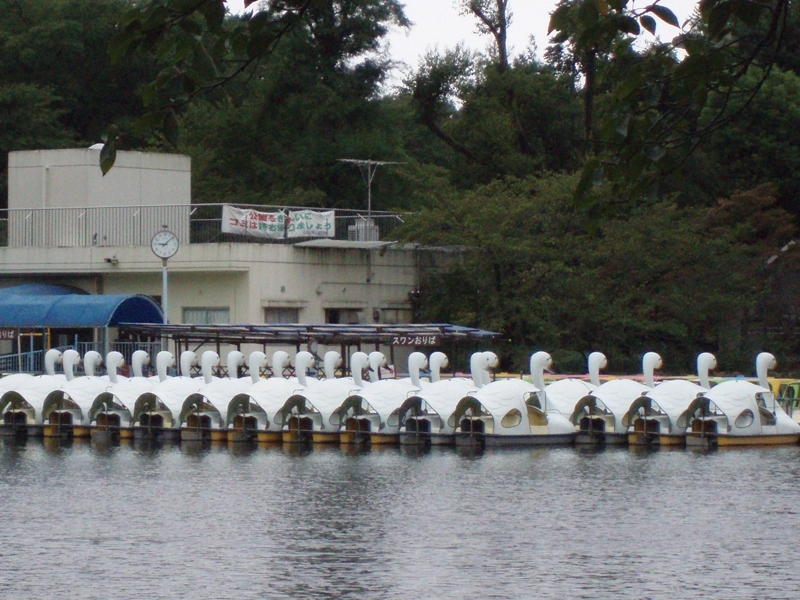This photograph likely depicts an early morning scene on a small lake in Asia, characterized by a row of approximately 20-25 white paddle boats each adorned with a large swan head in the front. These identical swan boats, typically rentals, feature a distinctive brown stripe and a seating area shaped like a swan's body. The water is calm and a steel-blue color, while the backdrop is dominated by lush green trees and a dark gray or off-white building, which serves as a rental station. Detailed with a blue awning extending from it and featuring a prominent clock indicating around 9:10 AM, the building also has a railing and possibly an antenna tower on its roof. A banner with red and green Asian characters hints at the location being in China or another Asian country. The serene setting is devoid of people, suggesting that it might be before the lake opens for the day's activities.